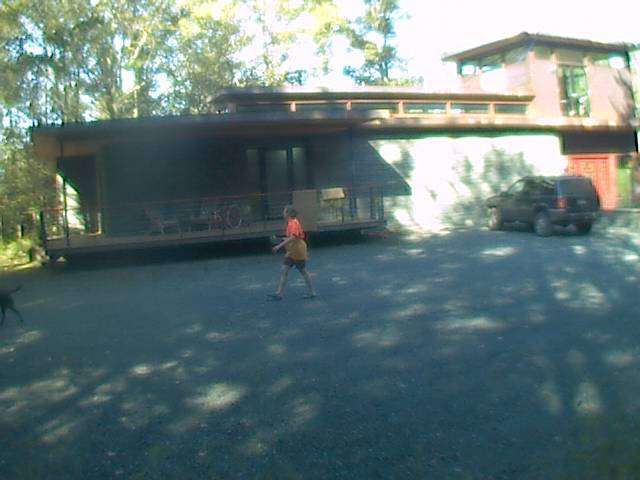A rustic home nestled in the wilderness. The house is styled like a large wooden cabin, surrounded by dense forest on both sides. The front of the home features a charming patio with four wooden rocking chairs neatly arranged. A woman is captured walking across the image, moving toward the left side of the frame, seemingly engaged in an unseen task. The scene exudes a tranquil, back-to-nature atmosphere.